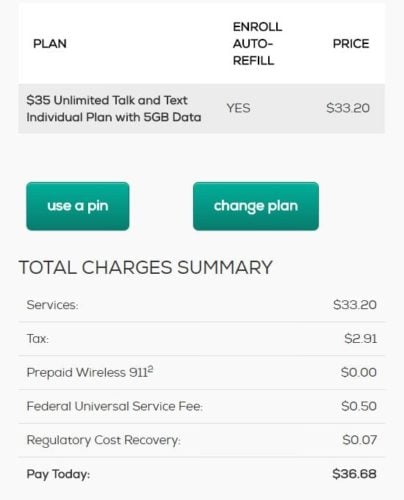This screenshot depicts a summary of a mobile phone plan with various details and charges. The plan includes unlimited talk and text, costs $35, and offers 5 GB of data for an individual line. The user is enrolled in auto-refill, which reduces the actual price to $33.20. 

Two green buttons are visible; one labeled "Use a Pen" and the other "Change Plan," both in white text. 

The total charges summary is also present, breaking down the costs as follows:
- Services: $33.20
- Tax: $2.91
- Prepaid Wireless 911: $0.20
- Federal Universal Service Fee: $0.00
- Regulatory Cost Recovery Fee: $0.07
- Total Pay Today: $36.68

The background of the screenshot is light gray, with a white section at the top.